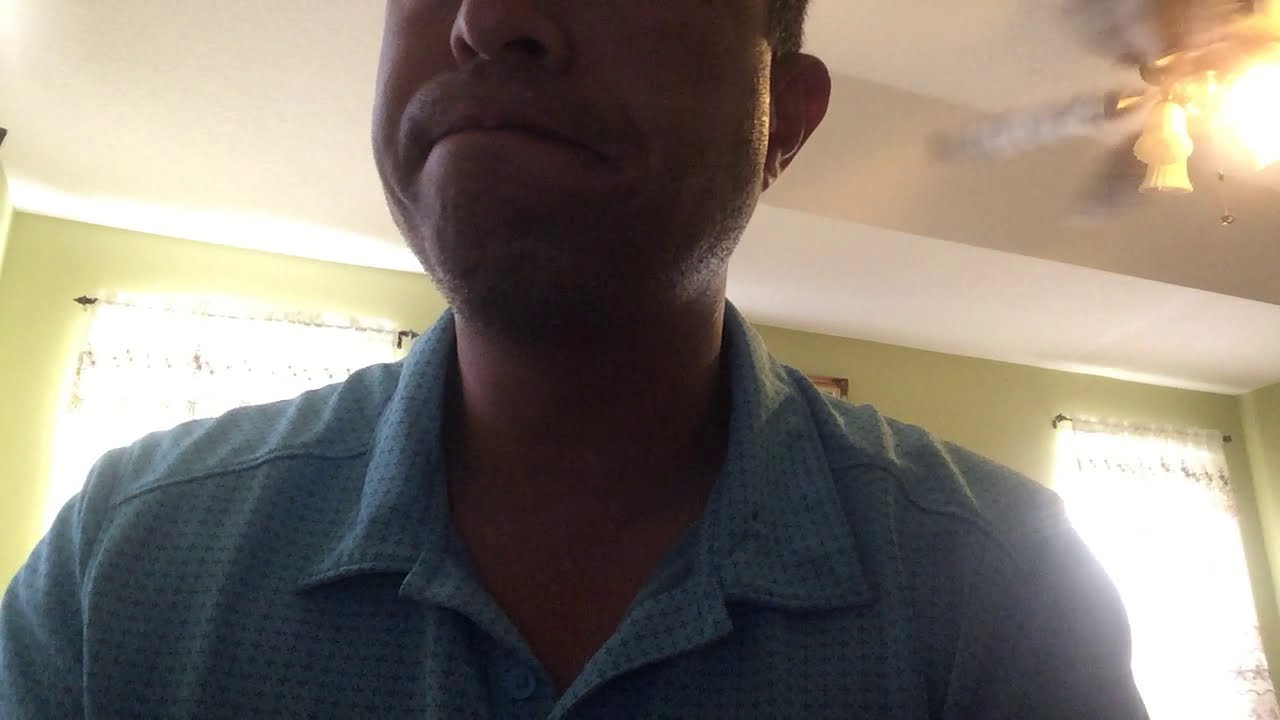This image features a close-up view of a Caucasian man in his 30s, captured from a slightly low angle that displays the lower half of his face to the upper third of his body. The man’s neutral yet concentrated expression gives the impression he is focused or perhaps resigned rather than angry, with his lips slightly pursed. He has a light stubble, indicating he hasn't shaved in a few days. He wears a light blue, button-up shirt adorned with fine checkered patterns that appear almost like a solid color from a distance.

His shoulders are positioned facing the camera, but his head is angled slightly to show his profile. The setting suggests an indoor environment with a white ceiling and greenish-yellow walls. The ceiling features a lit ceiling fan in motion, and there are sheer-curtained windows on the greenish walls allowing sunlight to filter through. Additionally, a ceiling fixture or light bulb is visible in the top left corner of the image. The overall ambiance of the room hints at a casual, slightly cluttered home setting.